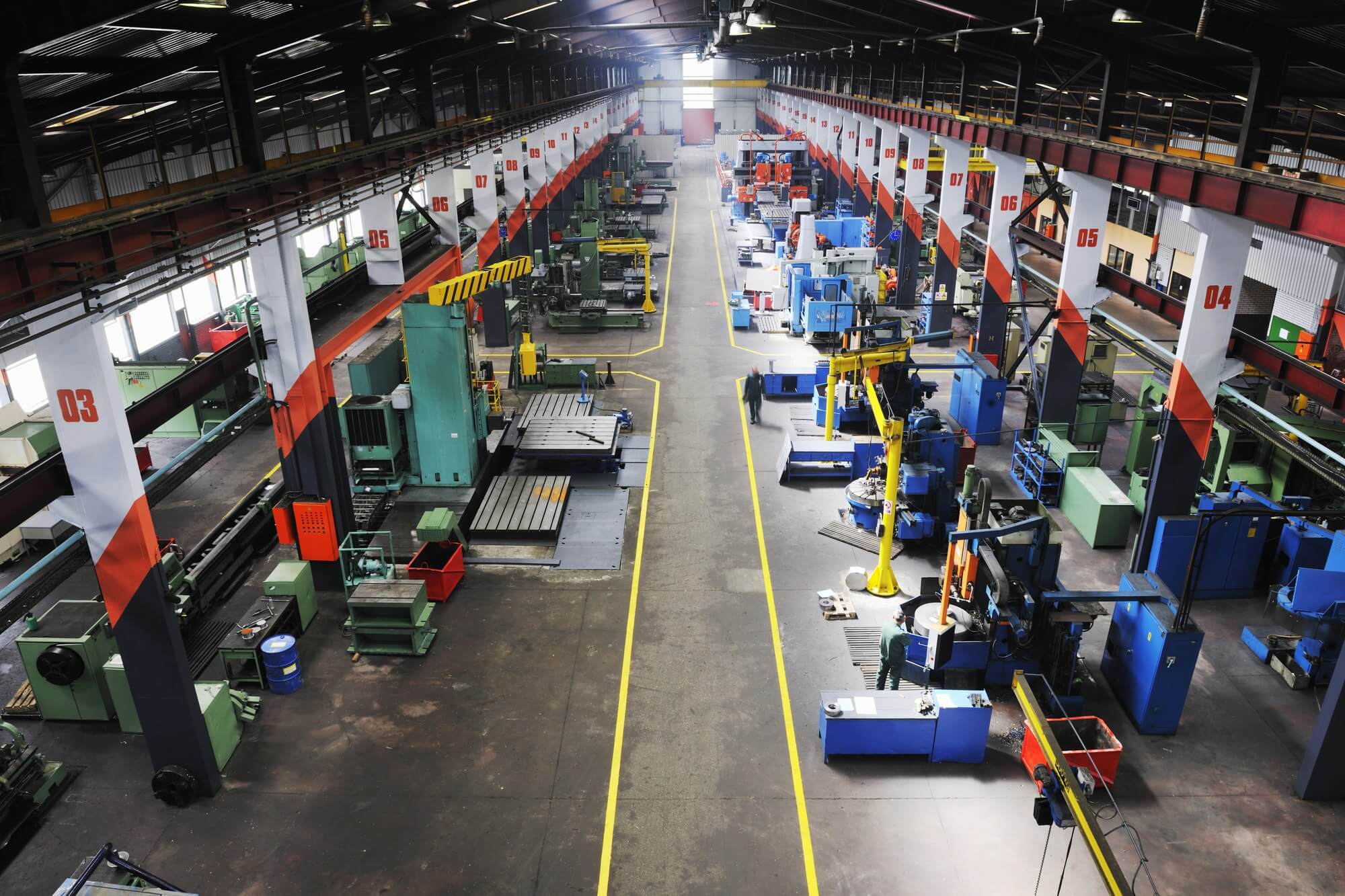The image captures the interior of a large warehouse or factory from an elevated vantage point, showcasing a steel-structured facility with a focus on its sprawling layout. The scene is characterized by a series of machinery scattered primarily along the left and right sides of a central aisle marked by a pair of yellow lines extending from the foreground to the background. The left side predominantly features greenish-blue equipment, while the right side is lined with blue machinery. Steel pillars support the upper levels, each decorated with black, red, and white stripes and sequentially numbered (03, 04, 05, etc.) starting from the left. The numbers and color bands help distinguish sections within the facility. Overhead, metal beams and cables are visible along with the metal ceiling, reinforcing the industrial atmosphere. The color palette within the image includes shades of gray, brown, yellow, blue, red, green, orange, white, and black, adding to the chaotic yet organized industrial setting.